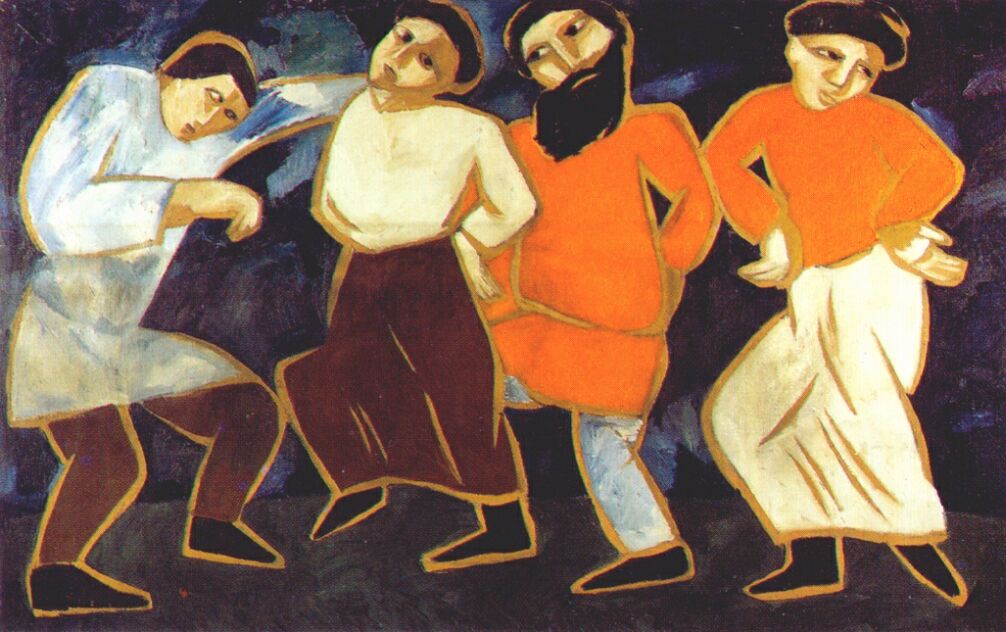The image portrays a vibrant, Picasso-like painting with four striking figures who appear to be dancing. Each figure has its own distinct attire and stance, contributing to the overall dynamic energy. 

On the left, a person in brown pants, a long white shirt, and black shoes wears an apron, possibly suggesting a working-class or artistic theme. Their head is tilted to the right, with their body facing forward but their legs directed to the side, highlighted with a yellowish outline, lending a dynamic twist to their posture.

Next to this figure is a woman in a long-sleeved white shirt and a brown skirt, also in black shoes. Her short black hair and head tilted to the right parallel the posture of her neighbor, enhancing the connection between the figures.

Moving rightward, a bearded figure in an orange shirt and what appears to be jeans stands out. Their dark beard and casual attire contrast sharply with the others, adding a textured depth to the ensemble.

The final figure, a female in an orange shirt and white skirt, also stands in black shoes. Her head is tilted to the left, forming a visual dialogue with the bearded figure. 

Behind this lively quartet, the abstract background features a melange of dark blue, light blue, purples, browns, and blacks, enhancing the scene’s artistic richness. Each figure's stance and attire, combined with the vibrant yet abstract background, creates a dynamic and engaging composition that captivates viewers.